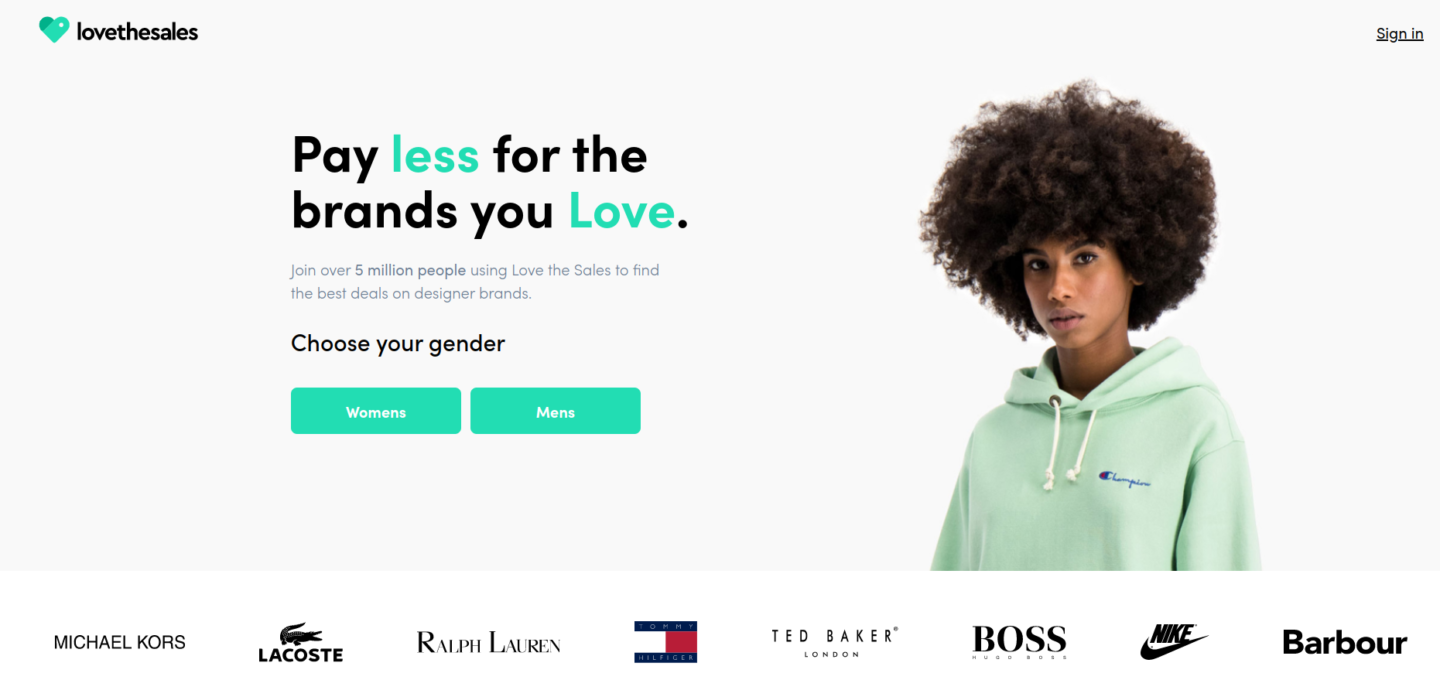The image showcases a web page for the company "Love the Sales." In the upper left corner, the company's icon and name "Love the Sales" are prominently displayed. On the upper right, a black-font link for "Sign In" appears against a white background.

In the middle of the upper section, a bold, inviting message is displayed: "Pay less for the brands you love." Here, "Pay for the brands you" is in black, whereas "less" and "love" are highlighted in blue. Beneath this, a smaller-font statement reads: "Join over 5 million people using Love the Sales to find the best deals on designer brands."

Below this message, a prompt to "Choose your gender" is followed by two blue buttons labeled "Women's" and "Men's," both with white font. To the right of these buttons is an image of a person wearing a mint-colored Champion hoodie.

At the bottom of the image, spanning from left to right, are logos of well-known companies including Michael Kors, Lacoste, Ralph Lauren, Tommy Hilfiger, Ted Baker, Boss, Nike, and Barbour.